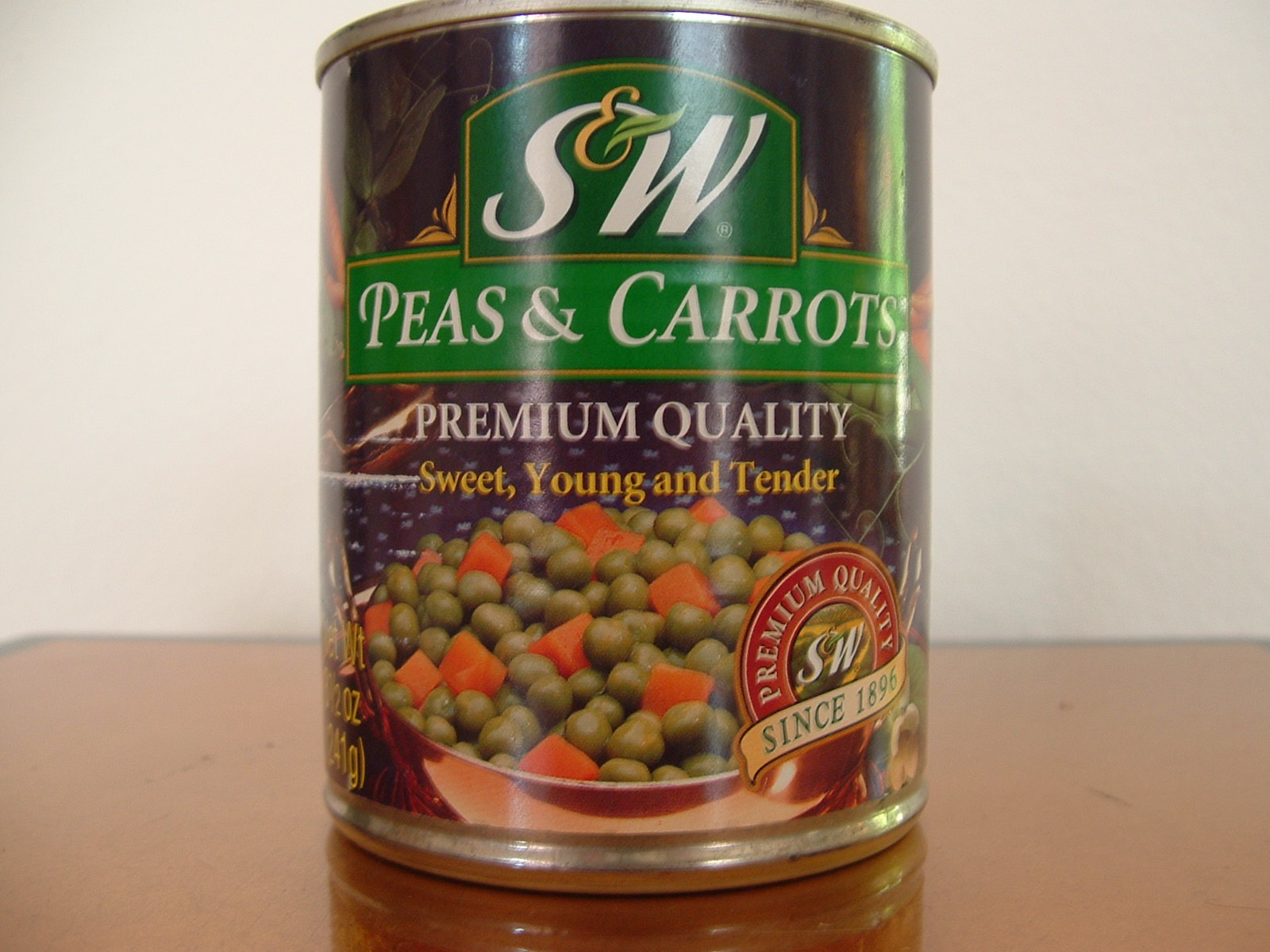This photograph features a can of peas and carrots. The label prominently displays "Peas & Carrots" in bold white text set against a green rectangle, which is accentuated by a thin gold border. Above this, there is another green rectangle with the brand "S&W" in white text, where the ampersand is rendered in gold and adorned with a small leaf. Below the brand name, the phrases "Premium Quality" and "Sweet, Young, and Tender" are printed, emphasizing the product's high standards and freshness. The label also includes a vibrant image of a bowl filled with colorful peas and carrots, illustrating the wholesome contents inside the can.